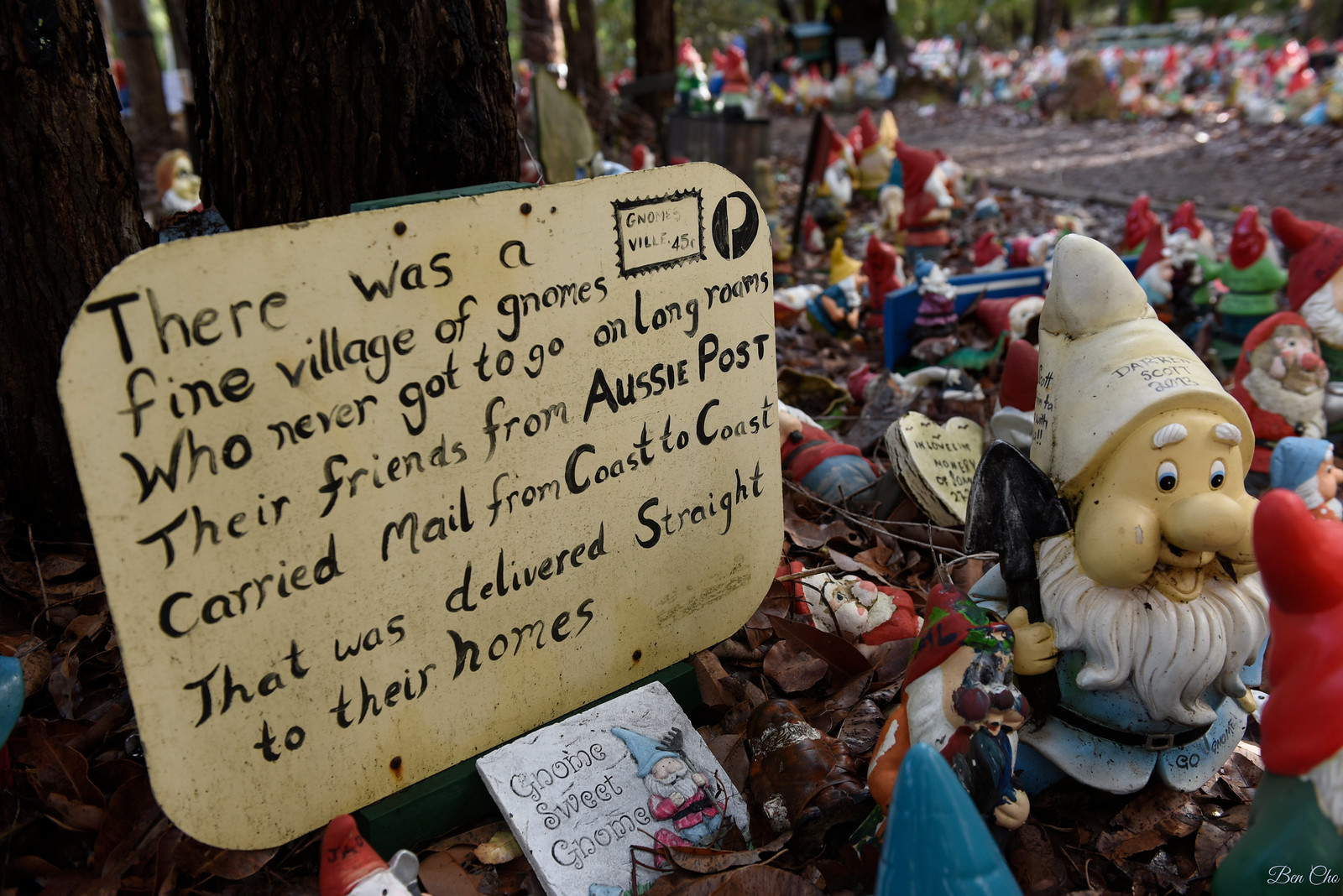This captivating outdoor photograph features a whimsical gnome village. Dominating the right-bottom area is a large gnome with a big white beard and a white hat, reminiscent of one of the dwarfs from "Snow White and the Seven Dwarfs." To its left, a tan sign with black letters stands out, reading, "There was a fine village of gnomes who never got to go on long roams. Their friends from Aussie Post carried mail from coast to coast that was delivered straight to their homes." A drawing of a stamp embellishes the top right corner of this sign, while a stone plaque below it reads "Gnome Sweet Gnome," featuring a gnome holding what looks like a spatula.

In the background, the photograph reveals a stunning assembly of dozens, if not hundreds, of gnomes arranged in rows, evoking a sense of endless continuity as they blur into the distance. These gnomes, some small and some large, are clad in old-fashioned Christmas attire with green outfits and red hats, giving a festive air to the scene. They appear to be resting on a bed of fallen leaves, adding a quaint, rustic charm to the display. This enchanting tableau offers a glimpse into a delightful, miniature world brimming with holiday spirit and imaginative detail.